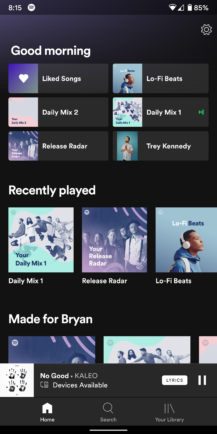This image, captured from a phone screen, showcases a user's music app interface. At the top, the screen welcomes the user with the text "Good Morning" prominently displayed in white font against a gradient background blending purples and blacks. Immediately below this greeting, there are six clickable sections labeled: Liked Songs, Daily Mix 2, Release Radar, Lo-Fi Beats, Daily Mix 1, and Trey Kennedy.

Proceeding further down the screen, there's a "Recently Played" section starting from the left with icons for Daily Mix 1, Release Radar, and Lo-Fi Beats. At the bottom of this section, a personalized category titled "Made for Bryan" (with "Bryan" spelled B-R-Y-A-N) is visible. Although the titles of the items in this personalized section are partially cut off, the visual icons suggest they correspond to Release Radar, Daily Mix 1, and likely Daily Mix 2.